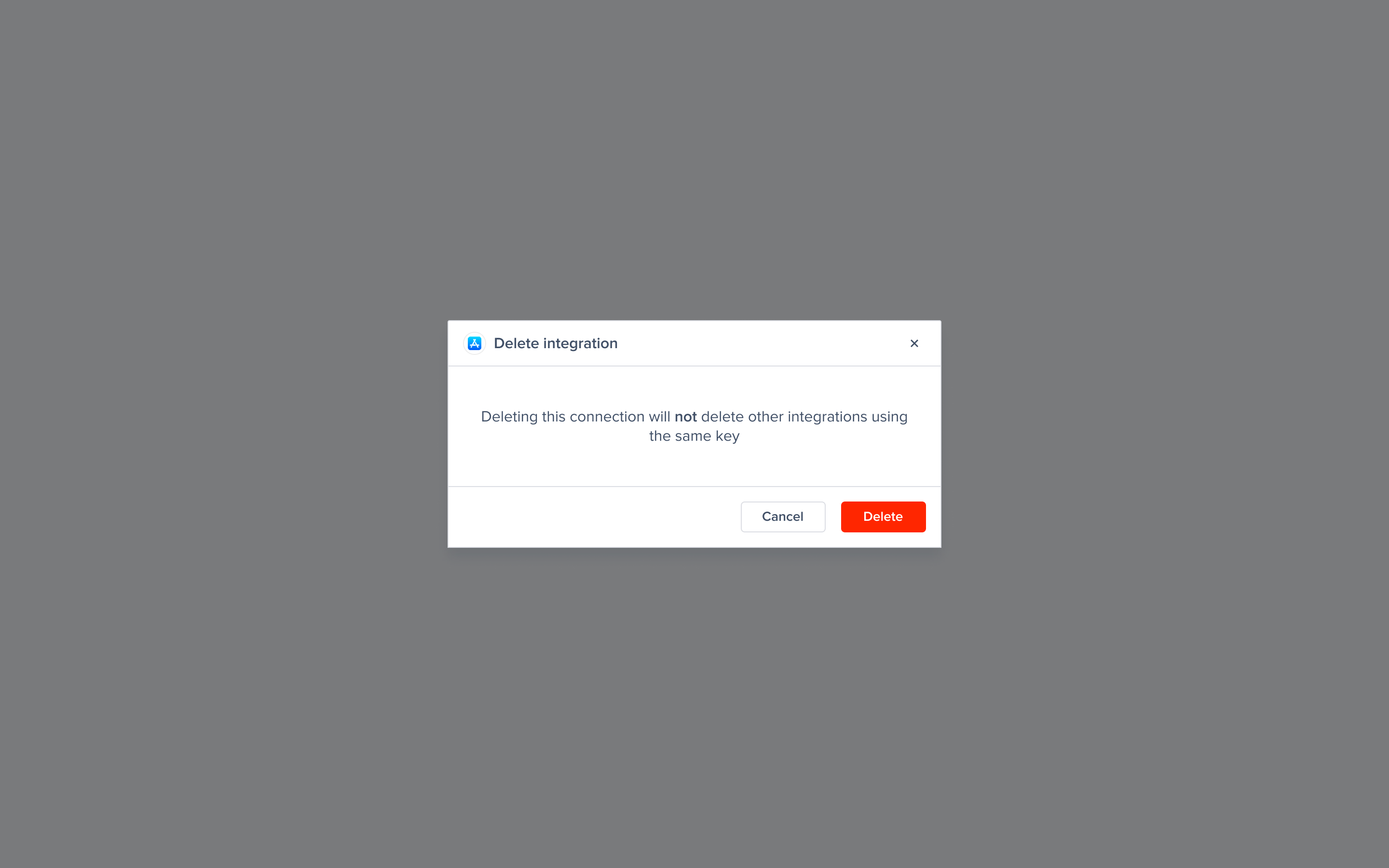The image depicts a screenshot of a computer screen, predominantly filled with a dark gray background. Centrally placed is a smaller white rectangle, which appears to be a pop-up dialog box. 

In the top left corner of this white rectangle, there is a tiny blue logo, barely legible due to its size. Adjacent to the logo, the text "Delete Integration" is prominently displayed. On the same line, in the top right corner, there is a small "X" icon for closing the dialog box. 

A light gray horizontal line separates the header from the main content of the box. Below this line, there's a message in black text that reads: "Deleting this connection will not delete other integrations using the same key." Another light gray line borders the bottom of the message.

At the bottom right side of the white rectangle, there are two buttons for user interaction: a white "Cancel" button with black text, and a red "Delete" button with white text. This minimalistic interface serves as a confirmation pop-up for deleting an integration, providing clear options and instructions for the user.